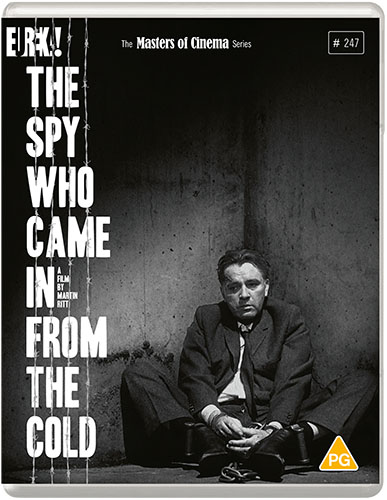The image, resembling the cover of a DVD or Blu-ray case, prominently features the title "The Spy Who Came in from the Cold" displayed vertically down the left side, one word at a time. At the top, the text "Eureka! The Masters of Cinema Series" is visible, along with the number 247. The background is an evocative black-and-white photograph of a man sitting on the floor in the corner of a dark concrete wall. He wears a black suit jacket and pants, and his expression appears ashen. A subtle detail shows metal objects, possibly chains, near his feet. The bottom right corner contains a yellow triangle with a white PG rating, and small text beside the word "in" credits the film to Martin Ritt. The overall aesthetic and design evoke a classic, vintage feel reminiscent of old VHS movie covers, with a white border adding a sense of depth to the case.